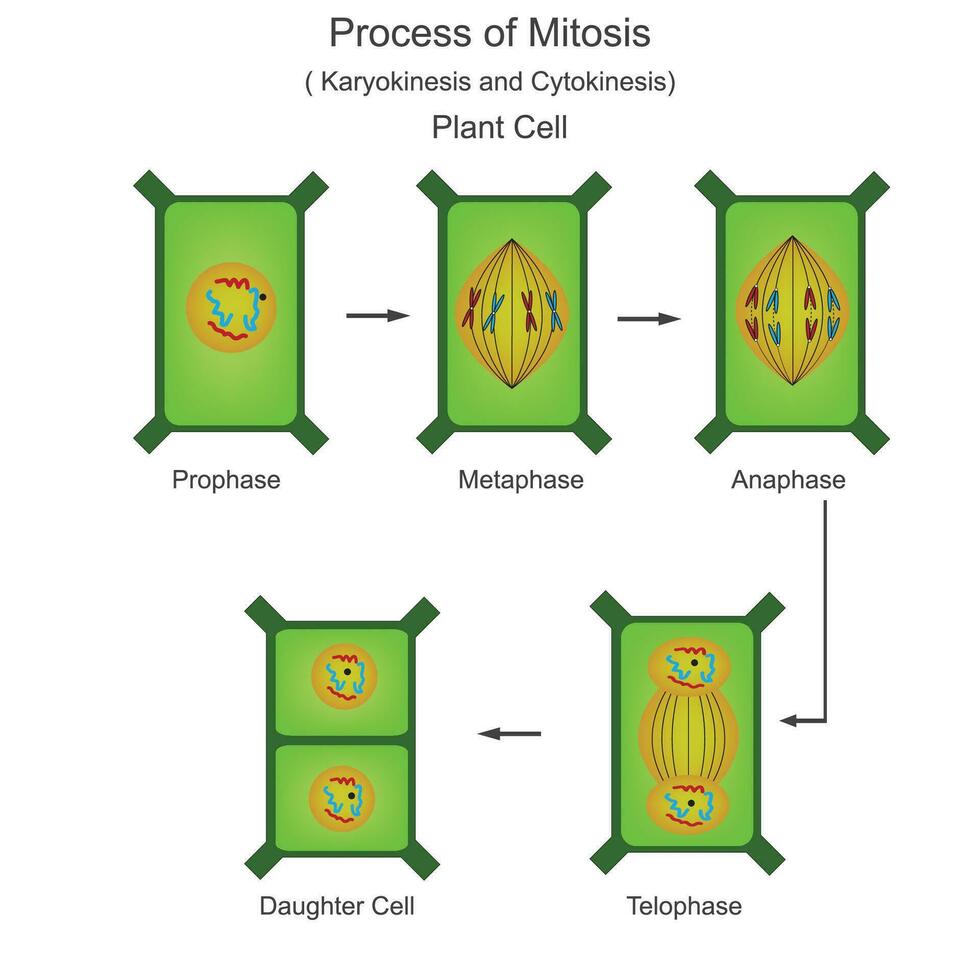This detailed scientific diagram illustrates the process of mitosis in plant cells, including karyokinesis and cytokinesis. At the top, in black text, it reads "Process of Mitosis (Karyokinesis and Cytokinesis) - Plant Cell." The diagram features five green rectangular boxes with dark green stubs at each corner, connected by arrows to indicate the sequential stages of mitosis.

1. The first box, labeled **Prophase**, shows a yellow circle containing red and blue squiggles, representing chromatin threads within the nucleus.
2. An arrow points to the second box, labeled **Metaphase**, depicting an elongated yellow oval (football-shaped) with red and blue X's, symbolizing chromosomes aligned at the metaphase plate.
3. Following this, an arrow directs to the third box, labeled **Anaphase**, presenting the same elongated yellow oval, but now the X's have separated into red and blue V's, indicating sister chromatids moving to opposite poles.
4. The next arrow points down to the fourth box, labeled **Telophase**, which shows a yellow circle split into three parts: the central part (future division site) and two circles at either end containing red and blue squiggles, representing the reformation of nuclei.
5. Finally, an arrow leads from Telophase to the last box labeled **Daughter Cell**. This box is divided into two parts, each containing a yellow circle with red and blue squiggles, symbolizing the two new cells, each resembling the original prophase stage.

Each visual element clearly delineates the transformation of the cell through each phase of mitosis, providing a comprehensive guide to understanding plant cell division.